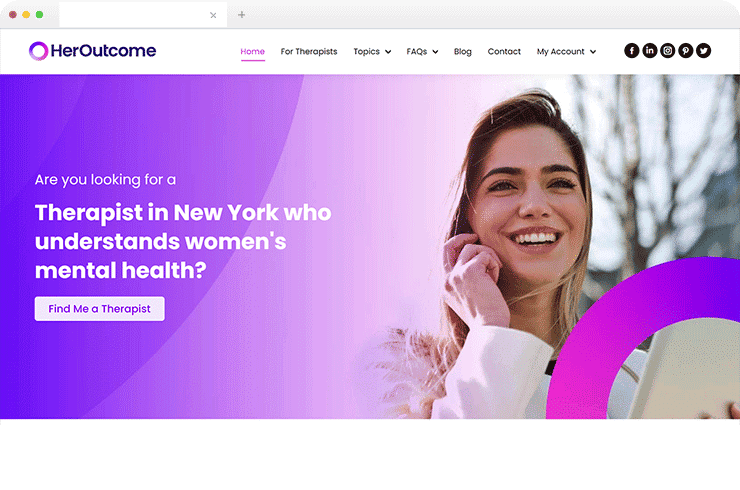**Detailed Caption:**

This is a screenshot of the homepage of the website "Her Outcome." At the top of the page, the website's logo features the name "Her Outcome" in deep purple letters. To the left of the name is a stylized zero, designed with multiple shades of purple and pink, forming a complete circle. 

To the right of the logo, a navigation bar features a sequence of buttons and links. First is a pink "Home" button. Following this are several options in black text on a white background: "Therapists," "Topics" with a pull-down menu, "FAQs" with a pull-down menu, "Blog," "Contact," and "My Account" with another pull-down menu. To the far right, there are icons linking to the website's social media pages on Facebook, LinkedIn, Snapchat, Twitter, and Pinterest.

The main image on the homepage showcases a brunette woman with blonde highlights, looking down at her phone or tablet, while smiling. She is dressed in light-colored clothing. The background of the image fades from a shade of pink on the right to a deeper purple on the left. Overlaying this gradient background, white text asks, "Are you looking for a therapist in New York who understands women's mental health?" Below this question is a button with gradient pink-to-purple text stating, "Find Me a Therapist."

Overall, this website appears to be a resource dedicated to helping women find therapists who specialize in women's mental health in New York.